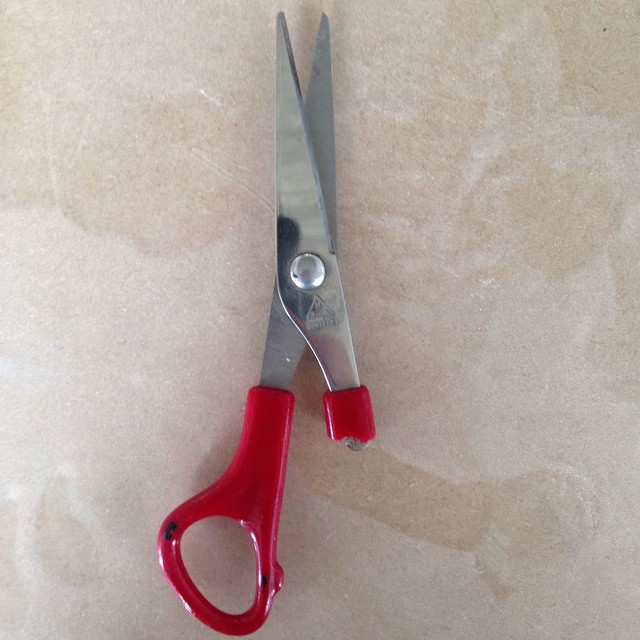This image features a slightly open pair of stainless steel scissors photographed from a top view against a textured beige background. The scissors, which are positioned with the blades pointing upwards, have one intact red plastic handle on the left, while the handle on the right is broken off, leaving only a small remnant. The background has a plush, velour-like appearance with several indentations. The remaining red handle shows some wear with small black marks, suggesting age. A subtle black reflection can be seen on the silver blades, possibly of the photographer.